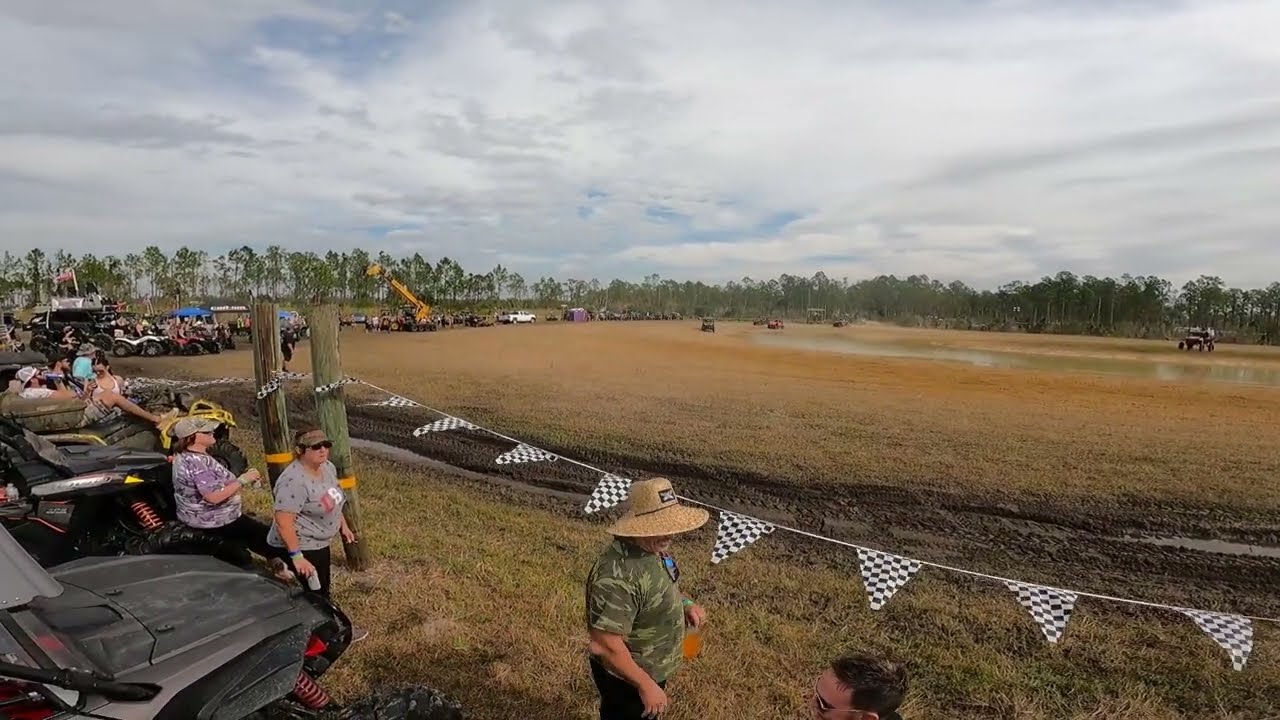The image depicts a dirt racetrack with a circular muddy track delineated by multiple logs driven into the ground, each strung with checkered flag streamers to mark the boundaries. Inside the track lies a green-colored pond surrounded by mud. Several off-roading vehicles, including four-wheelers and dune buggies, are parked around the edges of the track, with a few racing through the center. Spectators, including women in t-shirts and sun visors, and a man in a camouflage t-shirt and a large light brown bucket hat, are either sitting on their cars or standing nearby, watching the racing action. The scene is set against a backdrop of trees and an overcast, cloudy blue sky, with a yellow crane extended upwards visible in the distance.